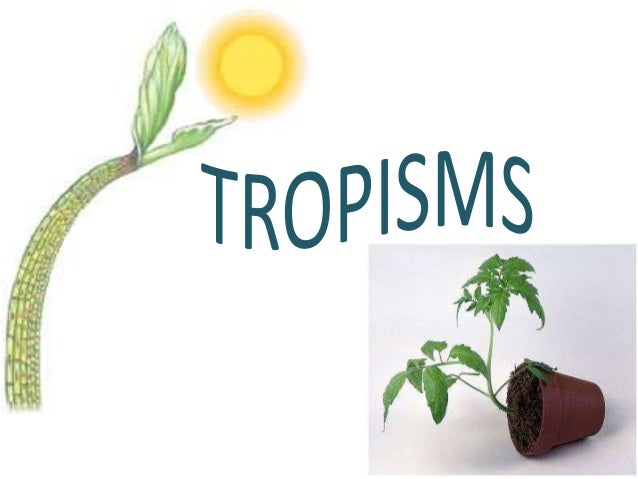The image appears to be a slide from a PowerPoint presentation with a white background, centrally featuring the word "TROPISMS" in wavy, dark teal or green letters. Positioned in the top left is a detailed, hand-drawn or digitally created illustration of a green plant stem with two leaves at the top, bending slightly to the right. Above this stem is a vibrant yellow sun with a golden ring. In contrast, the bottom right corner of the image displays an actual photograph of a toppled brown flowerpot on a light gray background. Despite the pot being on its side, the green plant remains rooted in the soil, with parts growing upwards toward the ceiling and parts lying flat. The scene showcases an interesting mix of digital art and real photography to illustrate the concept of tropisms. The colors used throughout the image include green, brown, yellow, orange, blue, and egg white.